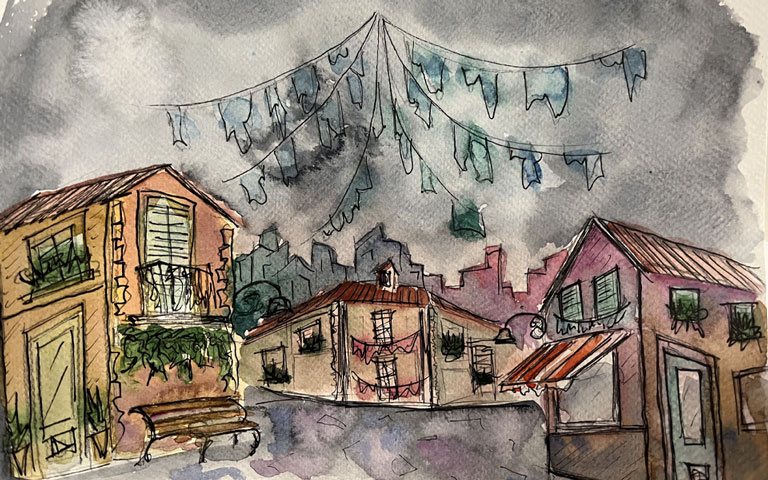This watercolor painting, framed in a horizontal rectangle, portrays an old cityscape with a blend of vibrant and muted tones. The scene features three prominent buildings set against a detailed background. On the left, there is a two-story house with a beige and pink hue, accented by planter boxes filled with green plants on the windows. Below, a brown bench rests in front of a pale yellow door, adding to the quaint charm. To the right of this house, the center stage is taken by a wider building, likely an apartment complex, adorned with red flags or perhaps lines of hanging clothes, stretched horizontally across it. The intricate details of the center building contrast with the city's gray-to-red skyline in the distant background. On the right side of the painting stands another structure, shaded in purple and beige, distinguished by a red and white awning over a bluish door. Above the entire scene, dark clouds fill the sky, and from a central point, green leaves or lines extend outward diagonally, adding a whimsical element to the somber atmosphere. The gray and white backdrop of tall high-rises enhances the painting's depth and evokes a sense of fading twilight.